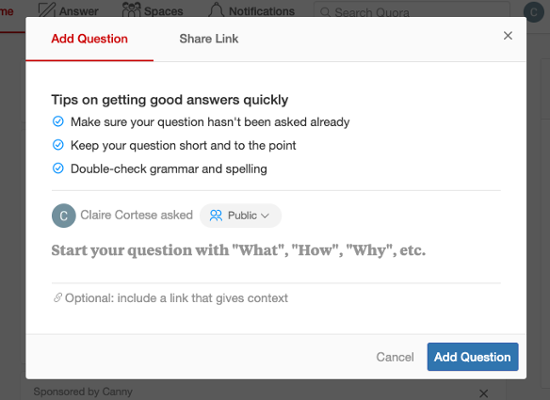The image is a screenshot of a menu on a mobile device displaying an "Add Question" interface. The interface presents several elements:

1. At the top, the text "Add Question" appears in red font, followed by "Share Link" in grey font on its right.
2. The user is currently on the "Add Question" tab, where it provides the heading "Tips on getting good answers quickly."
3. Under this heading, there is a list of three tips:
   - **First tip**: "Make sure your question hasn't been asked already."
   - **Second tip**: "Keep your question short and to the point."
   - **Third tip**: "Double-check grammar and spelling."
4. Beneath these tips, the text indicates that Claire Cortese has asked a question, which is set to the public privacy setting.
5. Additional guidance prompts users to start their question with words such as "what, how, why, etc." and suggests optionally including a link for context.
6. At the bottom of the interface, there are two buttons: a blue box labeled "Add Question" on the bottom right and a grayed-out "Cancel" button to the left of it.

All these elements are presented on a white background within a large white box. The rest of the screen, which appears to be the main part of the device's interface, is grayed out and not readable, emphasizing the "Add Question" menu.